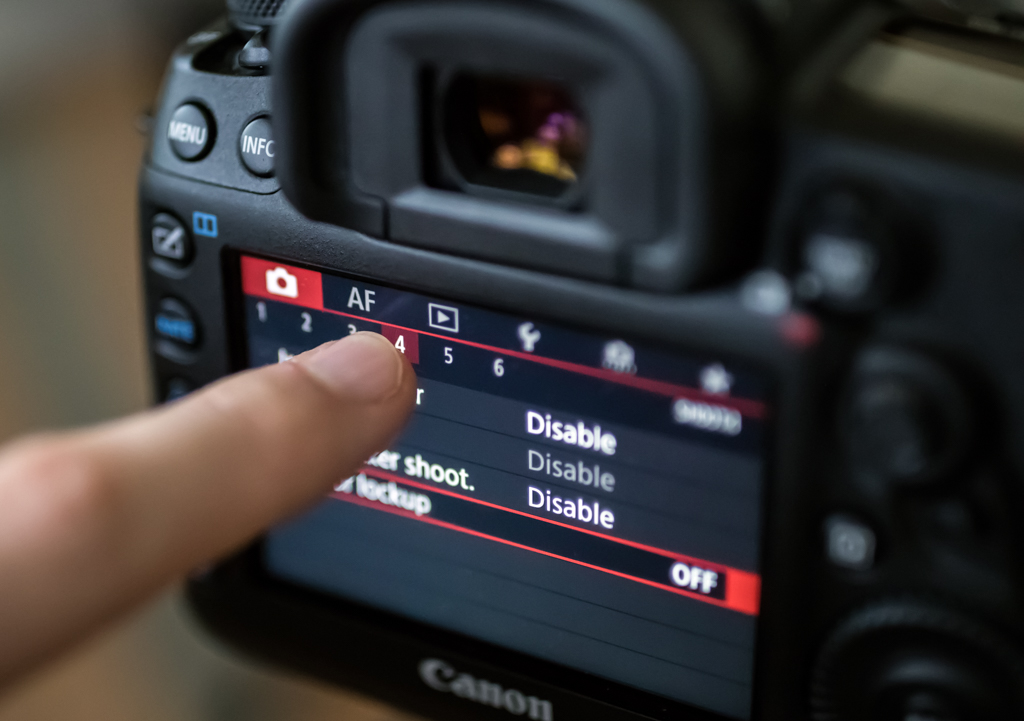The image captures a close-up of the backside of a black Canon digital camera. The camera’s digital display dominates the scene, showcasing various settings icons including options for AF, video, and tools, with three of the options labeled "disabled". The bottom option is highlighted in red and reads "off." A medium-toned finger, likely of a Caucasian individual, is tapping the screen, partially obscuring some of the labeled settings on the right side. The camera features various buttons like "menu" and "info," although many labels are blurred. The camera’s lens reflects some yellow and pink lights. The Canon logo is prominently displayed at the bottom of the camera base, and there are small blue emblems near the buttons. The background is blurry, emphasizing the close-up details of the camera itself.